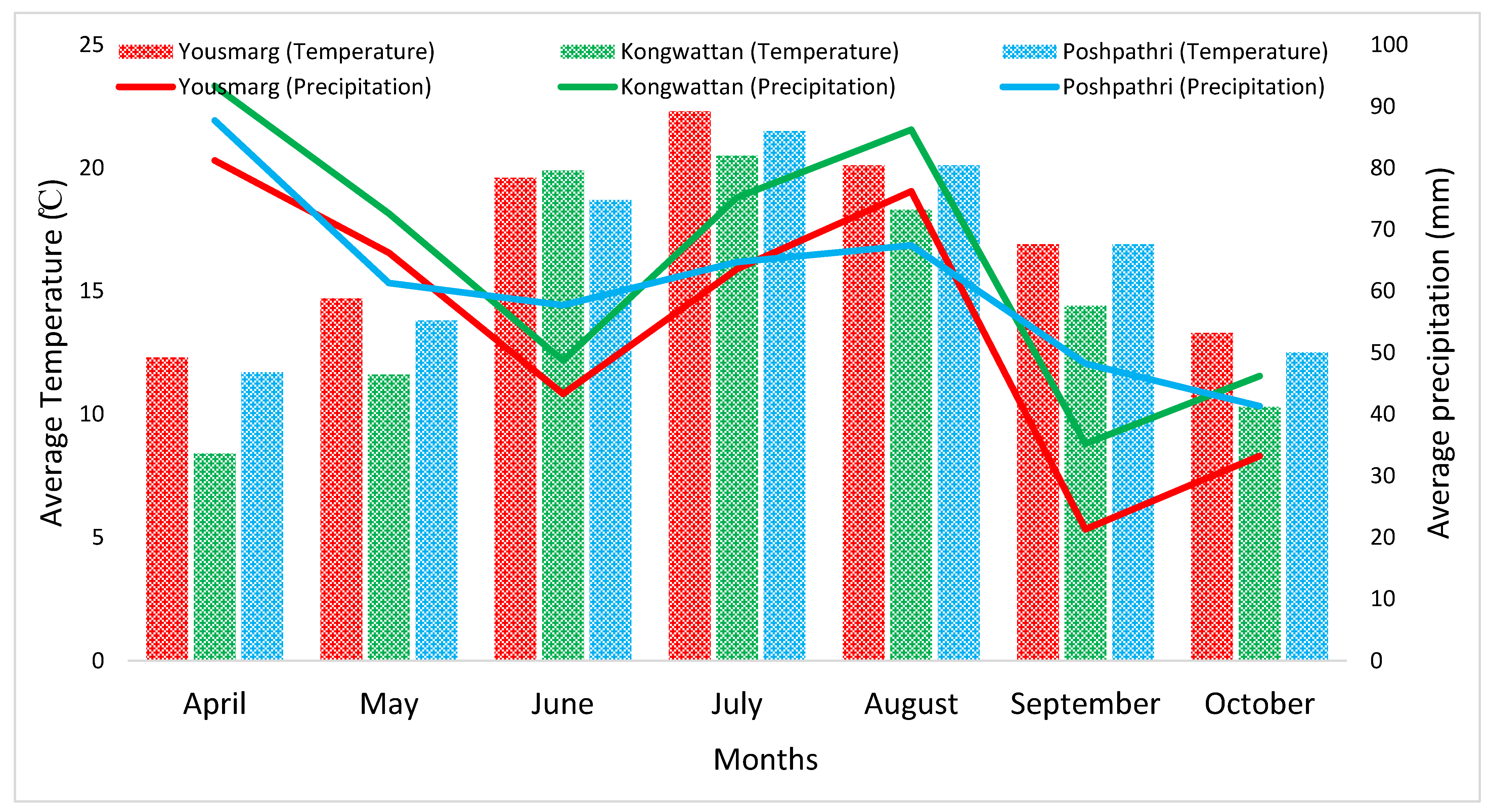The image shows a detailed bar and line graph comparing average temperatures in degrees Celsius and average precipitation in millimeters across three different locations: Yusmarg, Kungwattan, and Poshpathri. The graph spans the months of April through October. 

Temperature data is depicted with shaded bars in red for Yusmarg, green for Kungwattan, and blue for Poshpathri, while precipitation is represented by solid lines in matching colors. Along the left-hand side, the temperature scale ranges from 0 to 20°C, and along the right-hand side, the precipitation scale ranges from 0 to 100 mm.

The months are marked in normal black font along the bottom of the graph, with corresponding bars and lines above each month. The temperature trends show that Yusmarg consistently has the highest temperatures, followed by Kungwattan and Poshpathri, which fluctuate but generally align below Yusmarg. Precipitation trends, shown by the lines, depict varying patterns across the months.

A key at the top of the graph clarifies the color coding: shaded red for Yusmarg temperature, solid red for Yusmarg precipitation, shaded green for Kungwattan temperature, solid green for Kungwattan precipitation, shaded blue for Poshpathri temperature, and solid blue for Poshpathri precipitation. The graph is set against a white background with all text in black.